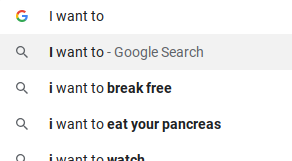The image depicts a screenshot of a Google search bar with autocomplete suggestions. The background is pristine white. At the very top, there is the iconic multi-colored "G" of the Google logo followed by the text "I want to" in dark black letters. Directly beneath, inside a light bluish-gray rectangle, a magnifying glass icon precedes the text "I want to - Google search" in black letters.

Further down, against the white backdrop, there are several autocomplete suggestions each beginning with a magnifying glass icon. The first suggestion reads, "I want to break free," with the phrase "break free" highlighted in bold. The subsequent suggestion reads, "I want to eat your pancreas," with "eat your pancreas" in bold. The final visible suggestion, which is partially cut off, reads "I want to watch," accompanied by the magnifying glass icon.